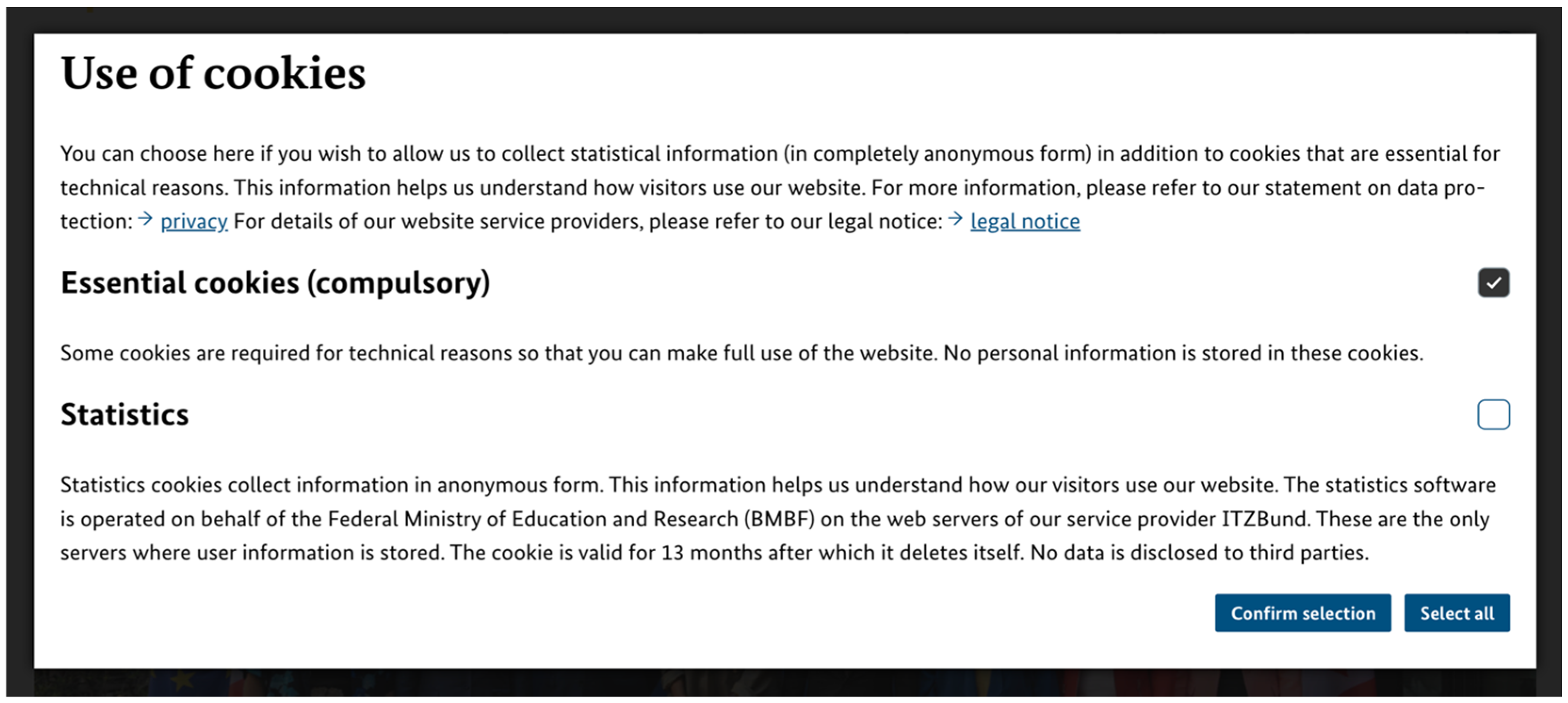Screenshot of a Cookie Consent Form on a Computer Screen

The image is a screenshot taken from a computer screen, showcasing a cookie consent form. The form is displayed inside a black-outlined rectangle. At the top left corner, the text reads "Use of Cookies." The main body of the form details the user's options regarding cookie preferences.

The initial paragraph explains, "You can choose here if you wish to allow us to collect statistical information (in completely anonymous form). In addition to cookies that are essential for technical reasons, this information helps us understand how visitors use our website." It also directs users for more information with the statement, "For more information, please refer to our statement on data protection. Privacy, for details of our website service providers, please refer to our legal notice."

Notably, the words "privacy" and "legal notice" are highlighted in blue, indicating clickable links.

Below this section, the form categorizes types of cookies:
1. Essential Cookies (compulsory): This section, marked with a checkmark, states, "Some cookies are required for technical reasons so that you can make full use of the website. No personal information is stored in these cookies."
2. Statistics: This section provides information on statistics cookies, stating, "Statistics cookies collect information in anonymous form. This information helps us understand how our visitors use our website. The statistics software is operated on behalf of the Federal Ministry of Education and Research on the web servers of our service provider, TTZ Bund. These are the only servers where user information is stored. The cookie is valid for 13 months after which it deletes itself. No data is disclosed to third parties."

At the bottom of the form, there are two buttons: "Confirm Selection" and "Select All," allowing users to make their cookie preferences known.